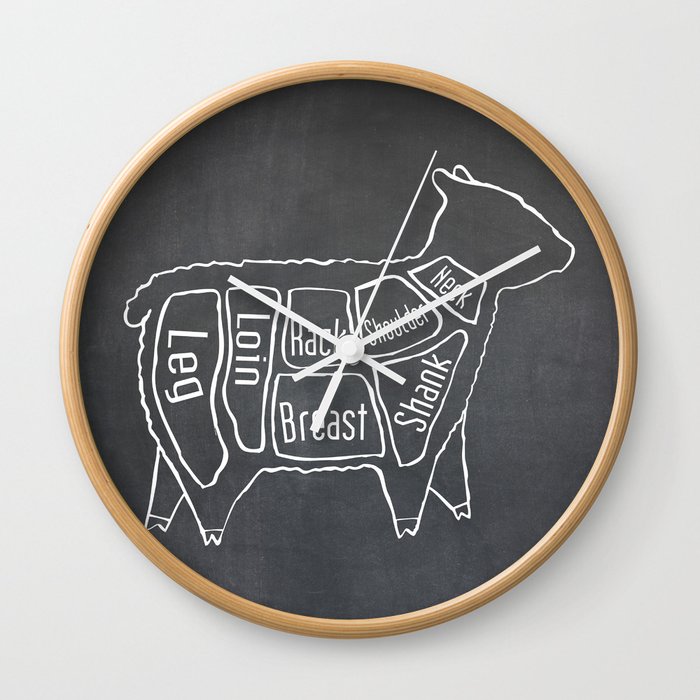The image shows a detailed photograph of a round wall clock prominently situated on a white wall, showcasing a modern interior decoration style. The clock features a distinctive wooden frame with a sleek, brown border, lending a contemporary yet rustic touch to the design. Its surface mimics a chalkboard texture, rendered in shades of gray and black. Most notably, the clock's face departs from traditional numeric markings and is adorned with a white, chalk-like outline of a cow. This outline is thoughtfully segmented and labeled with various parts of the cow, namely the neck, shoulder, shank, rack, breast, loin, and leg, resembling a butcher's diagram. The hour and minute hands are notable for their stark white color, standing out against the dark background, with the hour hand being slightly shorter. The clock is set to the time 10:10, adding a balanced aesthetic to the piece. This novelty clock blends functionality with visual intrigue, making it a unique piece of modern interior decor.